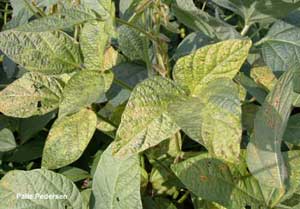The photograph showcases clusters of leafy green plants, with some flecks of pale yellow. The leaves are primarily green, with light green and darker green hues, and are heart-shaped with visible veins. Some leaves have small holes, suggesting they have been nibbled on by insects or affected by pests. The scene is illuminated by sunlight, casting natural shadows, indicating the image was taken outdoors during the day. The environment around the plants appears to be a garden or a natural park. There is a small white text at the bottom left corner of the image, but it is too small and blurry to be legible. The earth and dirt lie beneath the leaves, adding to the natural outdoor ambiance.